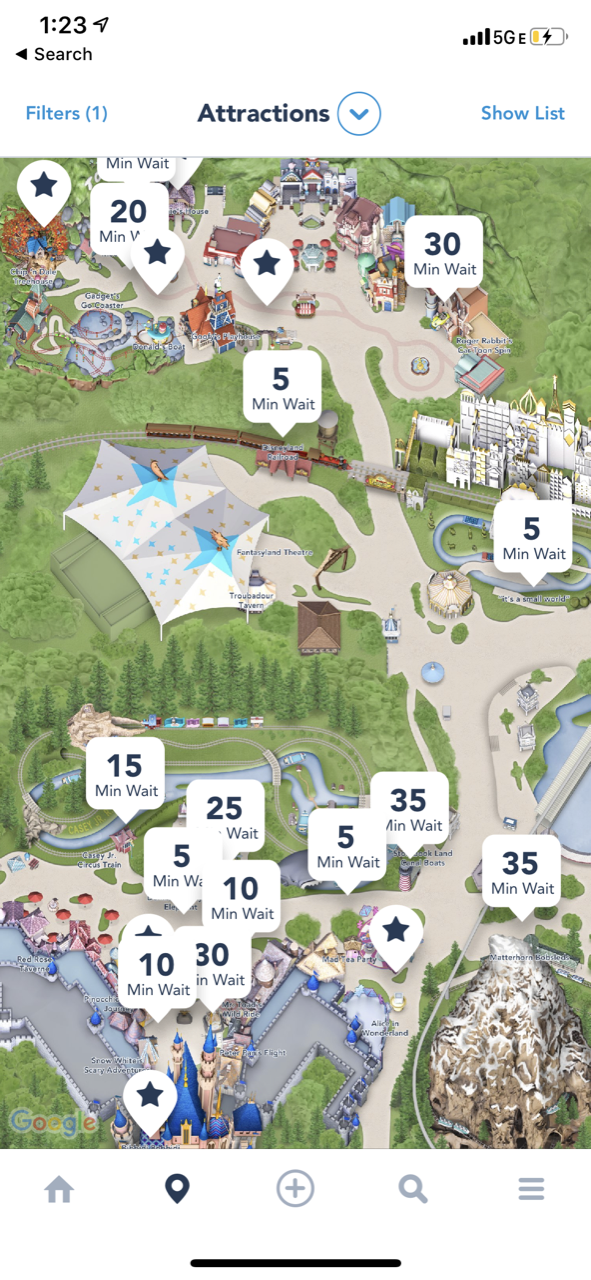The screenshot from the smartphone showcases various details. At the top of the image, the border is white with the current time displayed in dark grey font on the left side as "1:23" without specifying a.m. or p.m. Beneath the time, "Search" is written along with a left-pointing triangle icon. On the upper right corner, the indicators show a 5G network connection, a wireless signal icon, and a nearly empty battery that is currently charging, denoted by a small black lightning bolt.

In the center of the screen, the title "Attractions" appears on the left side, while options labeled "Filters" and "Show List," both in blue, are located on the right side.

The main part of the image features a relief map of an amusement park, rendered as a detailed drawing rather than a satellite image. The roads are illustrated in grey, green areas are displayed in green, and pine trees are depicted throughout the map. White squares with inverted triangle pointers indicate various locations on the map and provide information about wait times for different attractions. The wait times are displayed in large numbers followed by the abbreviation "min" for minutes and the word "wait." Various wait times are indicated, including 30, 35, 10, 5, and 20 minutes.